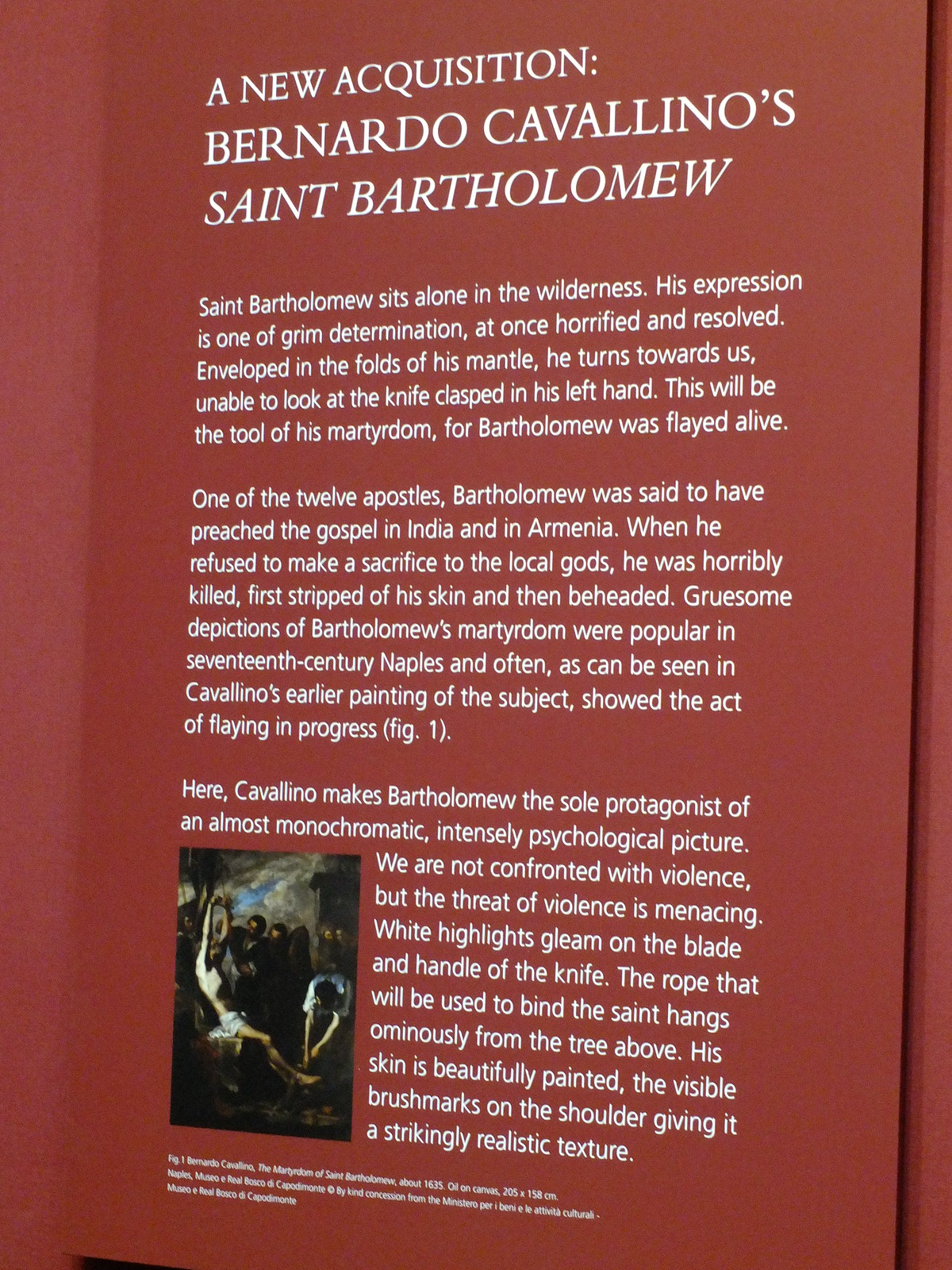The image shows an information poster presentation mounted on a reddish-brown wall, typical of a museum exhibit. The posterboard, also reddish-brown, prominently displays details in white text. At the top, large uppercase letters announce "A New Acquisition, Bernardo Cavallino's St. Bartholomew." Below, three intricately detailed paragraphs provide an in-depth account of the artwork. The description reveals the grim yet resolute expression of St. Bartholomew, one of the twelve apostles, who met his end through flaying and beheading for refusing to renounce his faith. Cavallino’s painting captures Bartholomew alone in the wilderness, enshrouded in melancholic folds, his face turned away from the knife in his hand—a symbol of his imminent martyrdom. The text describes how the painting, rendered in an almost monochromatic palette, evokes a powerful psychological tension without direct violence, highlighting Bartholomew as the central figure amid an ominous atmosphere. In the lower left corner of the poster, a small image of the artwork illustrates these elements: Bartholomew bound, with other shadowy figures around him, enhancing the narrative of his suffering and resolve. Beneath this image, further text continues in white but is difficult to read from a distance.